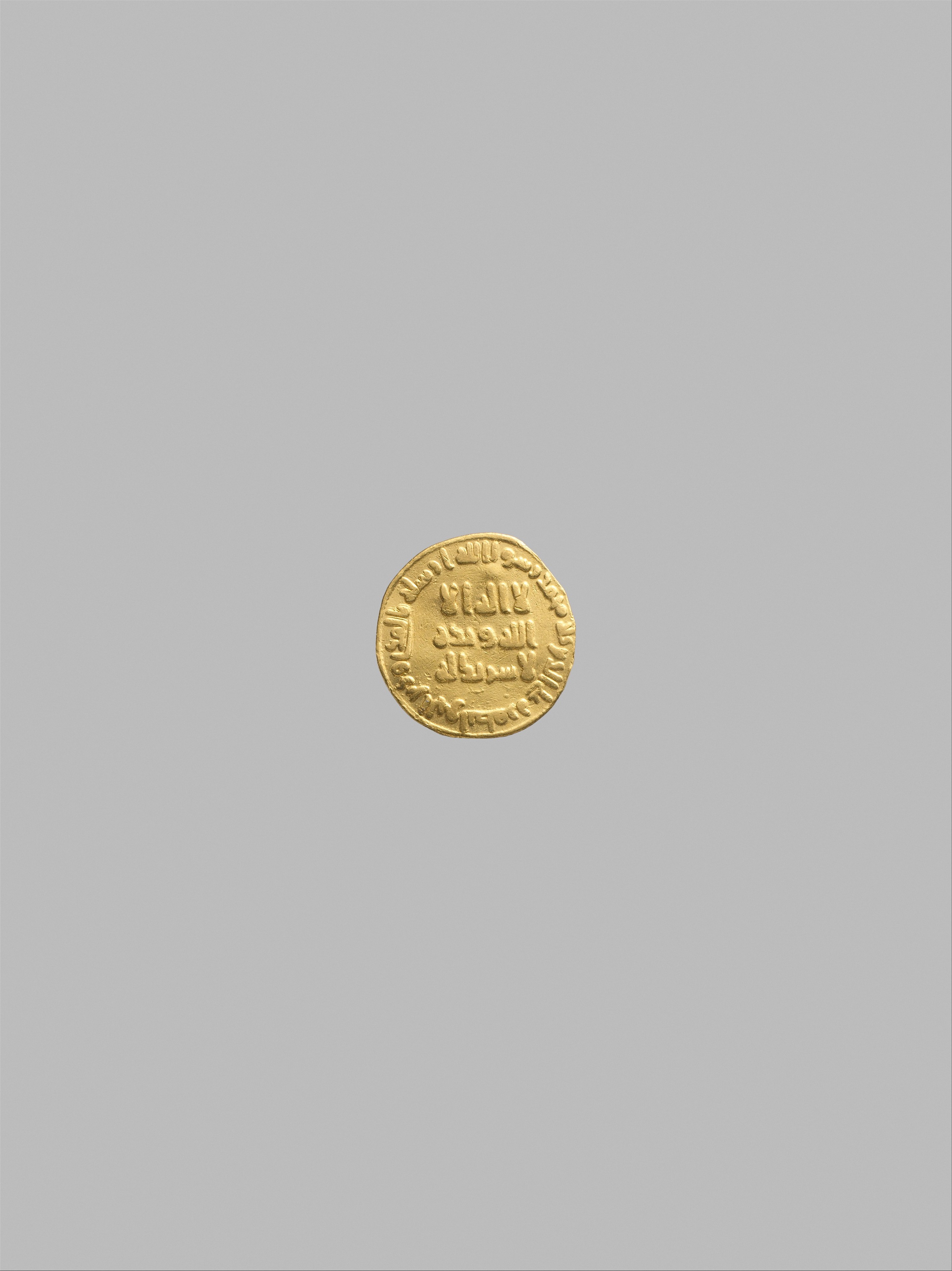The image showcases a golden, ancient coin against a light gray background, appearing almost as if it were scanned. The coin is round but slightly misshapen with visible imperfections and a slight lip around the rim. It features etchings and raised, embossed lettering in an ancient language along the border and in the center. Despite not being able to identify the specific language or country of origin, the coin appears well-preserved with no signs of deterioration. The overall lack of shadow and dimension suggests this could be a flat, cropped image of the coin's front side.